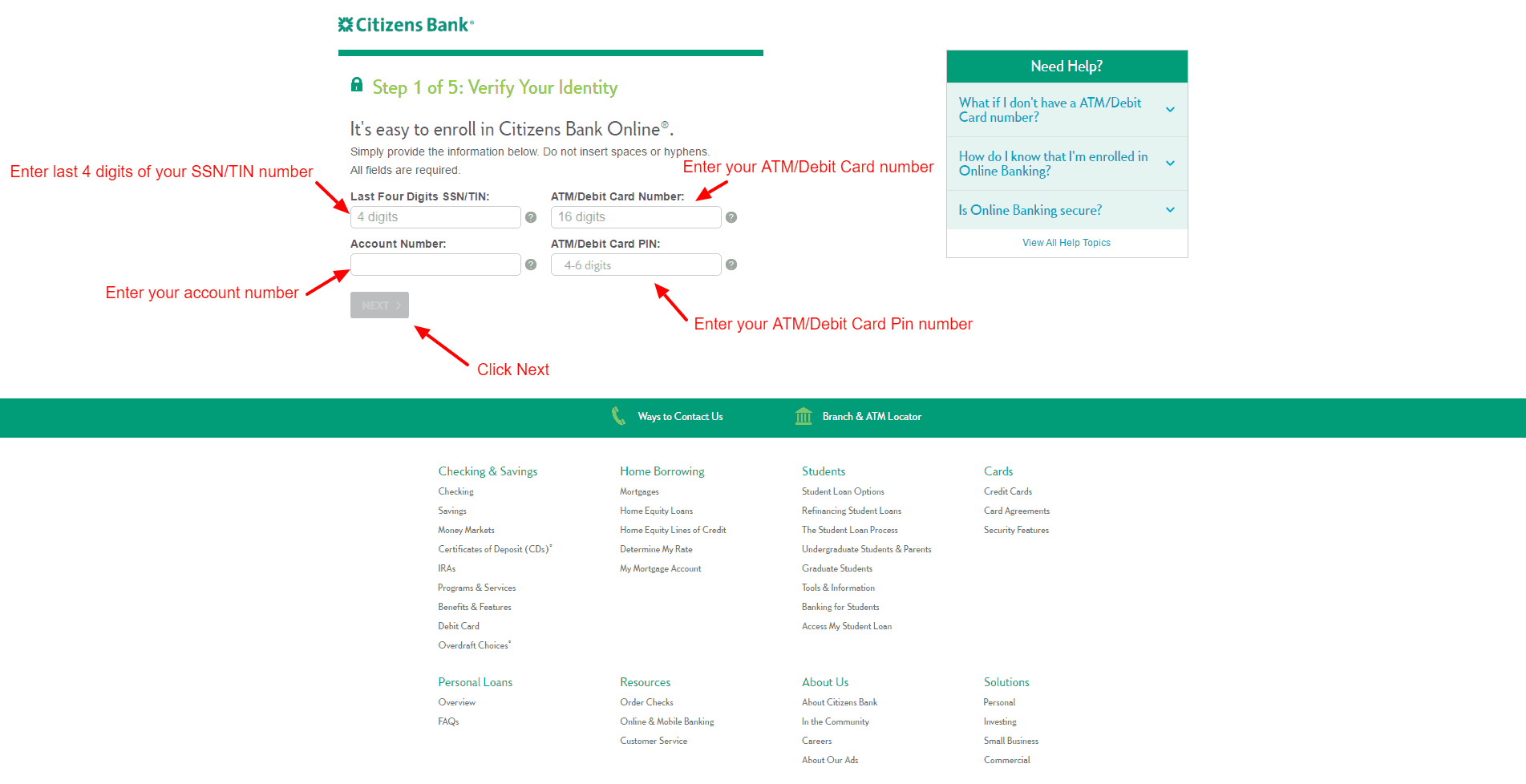The image displays a Citizens Bank web page designed for online account enrollment. At the top, the Citizens Bank logo is presented in green, followed by a green line. Below, the page indicates "Step 1 of 5: Verify Your Identity." The text beneath in black reads, "It's easy to enroll in Citizens Bank online," followed by smaller, less readable print.

Several instructional arrows guide the user through the process:
- The top left arrow prompts to "Enter the last four digits of your SSN/TIN number."
- To the right, another arrow directs users to "Enter your ATM debit card number."
- Below these instructions, users are asked to "Enter your account number."
- An additional step involves clicking "Next" and entering your "ATM debit card PIN number."

To the right, under a green label reading "Need Help," there are additional unreadable instructions likely to assist users who do not have an ATM debit card or who encounter other issues.

At the bottom of the page is a green bar with links to various sections of the website, including "Checking and Savings," "Students," and "About Us," among others. However, some of the text appears too small to read clearly.